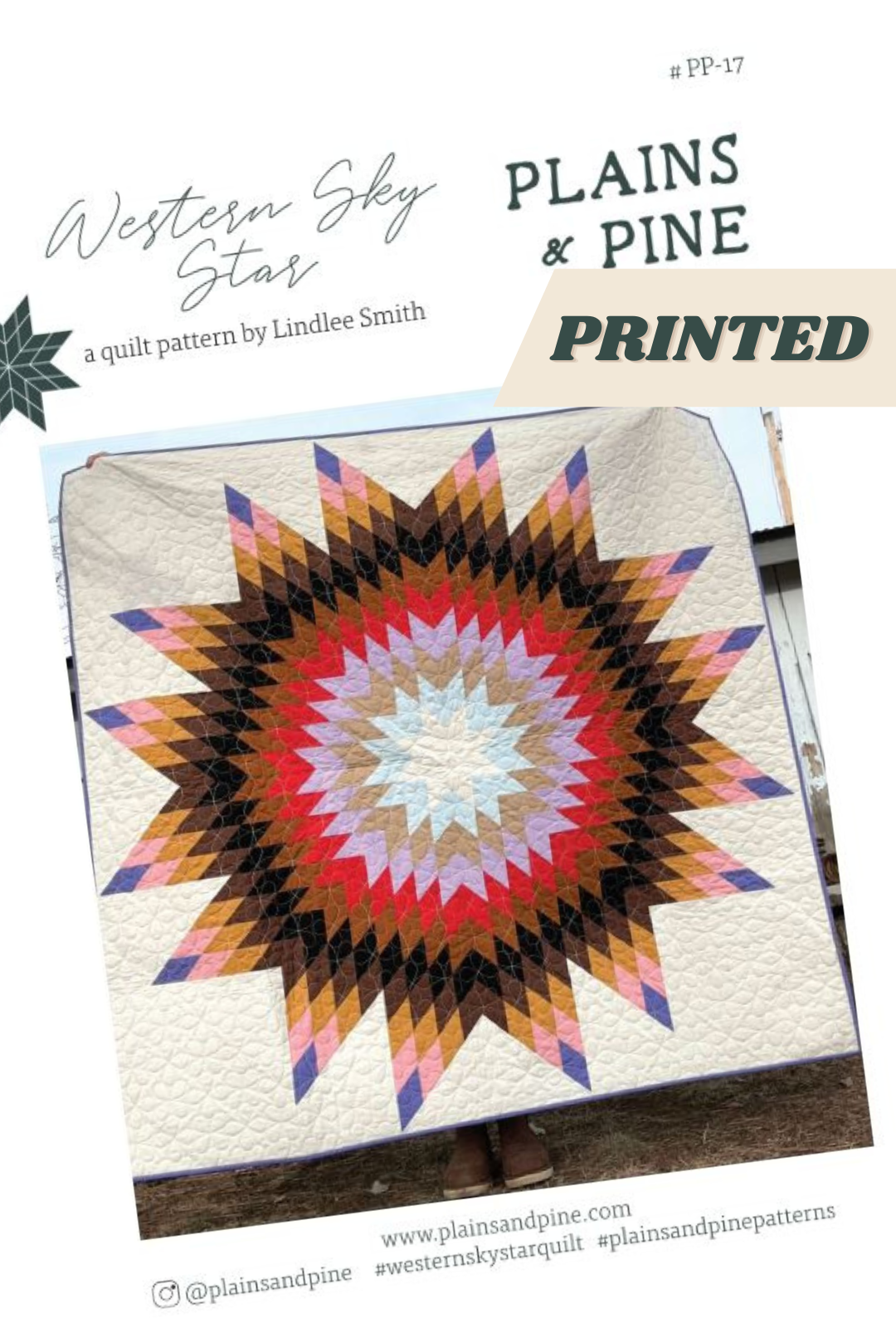The image features an advertisement for a quilt pattern titled "Western Sky Star" by Lindley Smith, showcased on what appears to be a magazine cover with a white background. Prominently displayed in the center is the quilt, which exhibits a striking sunburst or starburst design. The intricate pattern begins with a white core, transitioning outward through shades of light blue, brown, purple, red, and several layers of brown, culminating in spiky triangular points at the edges. The design creates a dynamic, multi-colored star effect. The advertisement includes the website www.plainsandpine.com and their Instagram handle, Plains and Pine, along with additional company information. The quilt itself is held up by an individual, with their shoes barely visible beneath it, standing on a brownish carpet.